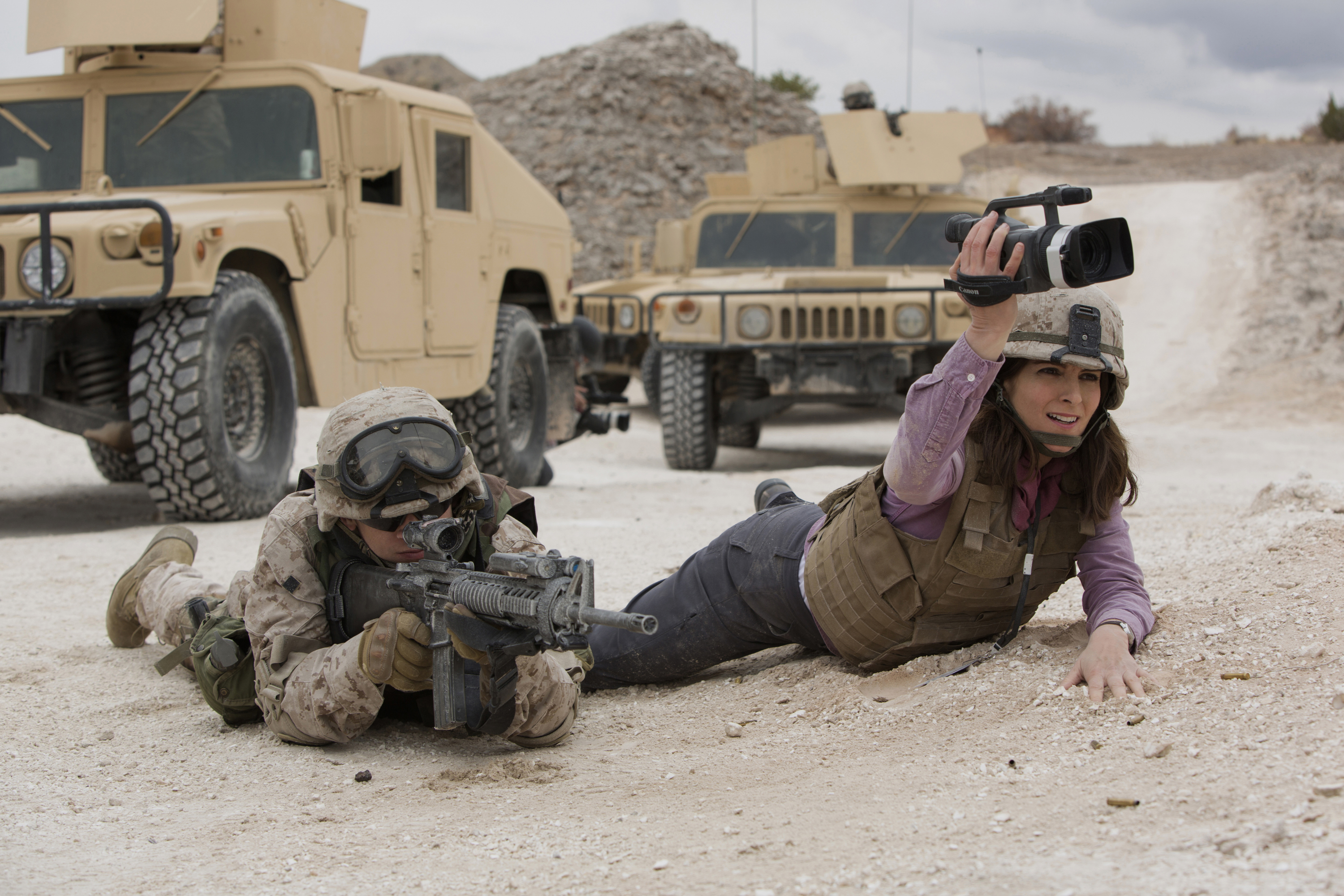The photograph is a horizontally oriented, rectangular image capturing a military scene possibly from Iraq or Afghanistan. Dominating the foreground on the left, a soldier is in the prone position aiming through the scope of his black assault rifle. He is dressed in desert-colored camouflage with tan and brown spots, complemented by a forest-green and brown camouflage combat vest. His helmet, which is adorned with black goggles, and multiple pouches on either side, enhance his tactical readiness. He wears brown boots and gloves, adding to his rugged appearance.

To his right, a photojournalist lies on her stomach, capturing the action with a black handheld camera held above her helmet. She is dressed in a purple long-sleeve shirt, black jeans, a brown bulletproof vest, and a similar army green helmet. Her long brown hair cascades beneath the helmet, highlighting her intense focus on documenting the scene.

In the background, the image captures two to three Humvee military vehicles positioned on a light brown, sandy dirt road interspersed with gray rocks. These low-slung vehicles are equipped with black tires, light brown armored metal bodies, and prominently feature turret guns on their roofs protected by metal guards. The area is scattered with rubble, sparse patches of grass, and dusty, sandy terrain, painting a vivid picture of a war zone in action.